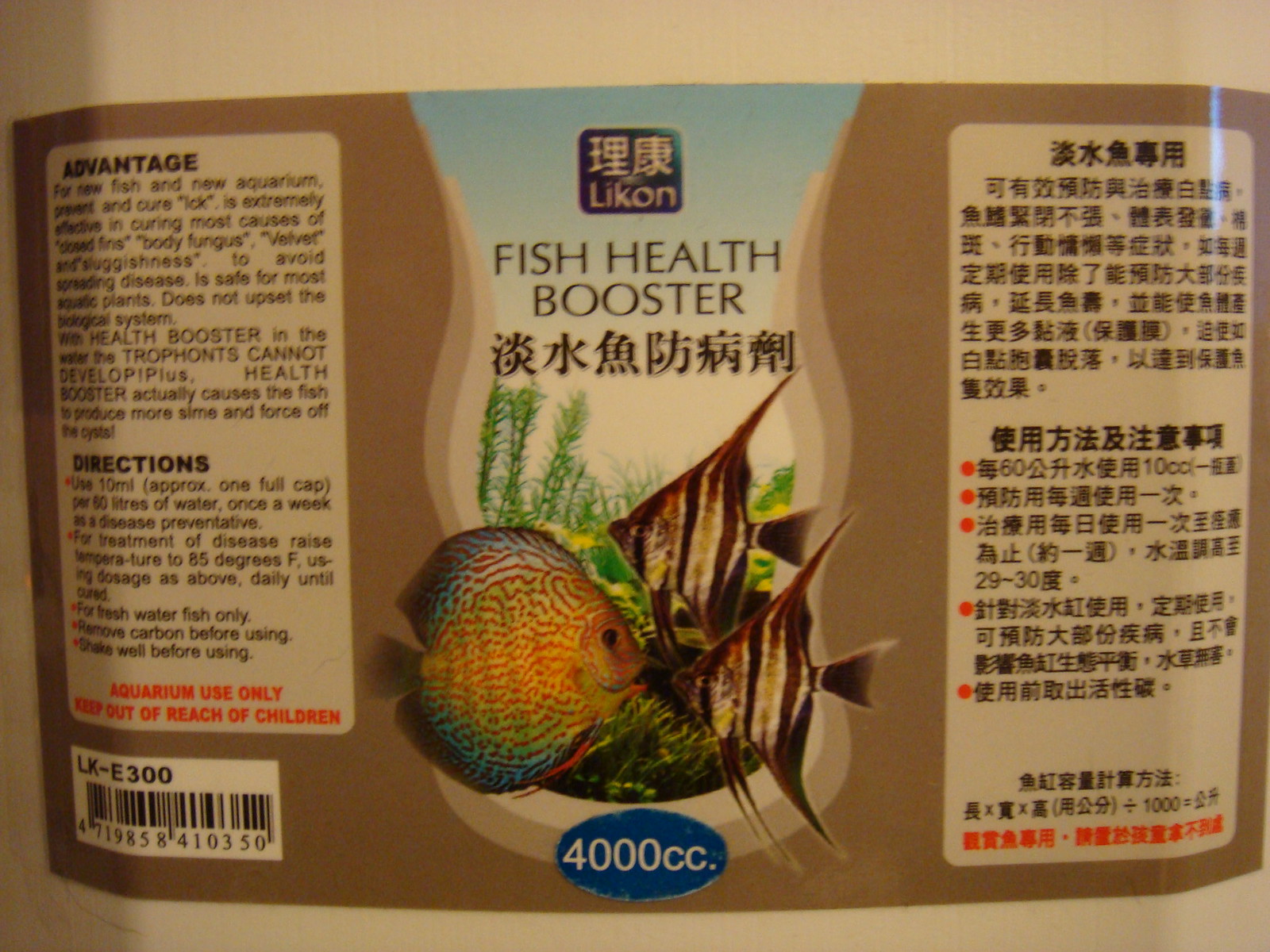The label on the bottle is a detailed fish health booster product, likely an Asian import or foreign-made item produced by Likon. The bottle itself has a beige-white color, with a slightly darker beige label. At the top of the label, "Fish Health Booster" is prominently displayed, followed by the same title in Chinese characters.

Beneath the title, there's a vibrant image of a blue and orange fish facing right, accompanied by two striped angelfish facing left, creating a visually engaging scene. The background of the image includes green vegetation and seaweed, enhancing the aquatic theme. Below the fish, the text "4000 cc" is written in white letters within a blue oval.

On the left side of the label, there's an information panel starting with the heading "Advantage," followed by a explanatory paragraph, and then "Directions" with usage instructions. At the bottom left corner, the UPC code is displayed. The right side of the label mirrors this information in Chinese characters. The product claims to be beneficial for new fish and aquariums, safe for most aquatic plants, and does not disrupt the tropical ecosystem. The usage instructions suggest adding a full cap of the product to the water.